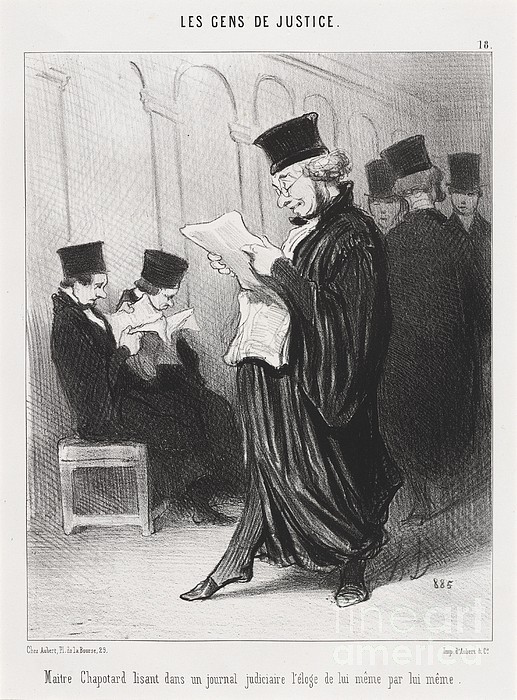The image is a vintage black-and-white comic illustration titled "Lessons to Justice," depicting a scene in a courtroom. At the center, an older man with a beard and glasses, dressed in formal attire including a long black coat and a hat, is engrossed in reading a white newspaper. Surrounding him are five other men, making a total of six, all similarly dressed in formal black coats and hats. Two men are seated on a bench to the left, also absorbed in reading newspapers, while three others in the background are engaged in a discussion. The courtroom setting is detailed with period-specific attire, including large narrow-brimmed caps, stockings, and black shoes. The comic includes text at the top and bottom, written in an old-fashioned font, with French phrases like "module chapter listed dense and journal" and "Luna men parliament." The number 18 is visible in the top right corner, suggesting the comic might be part of a series or publication sequence. The detailed pencil artwork captures the essence of a judicial and legislative environment from a bygone era.